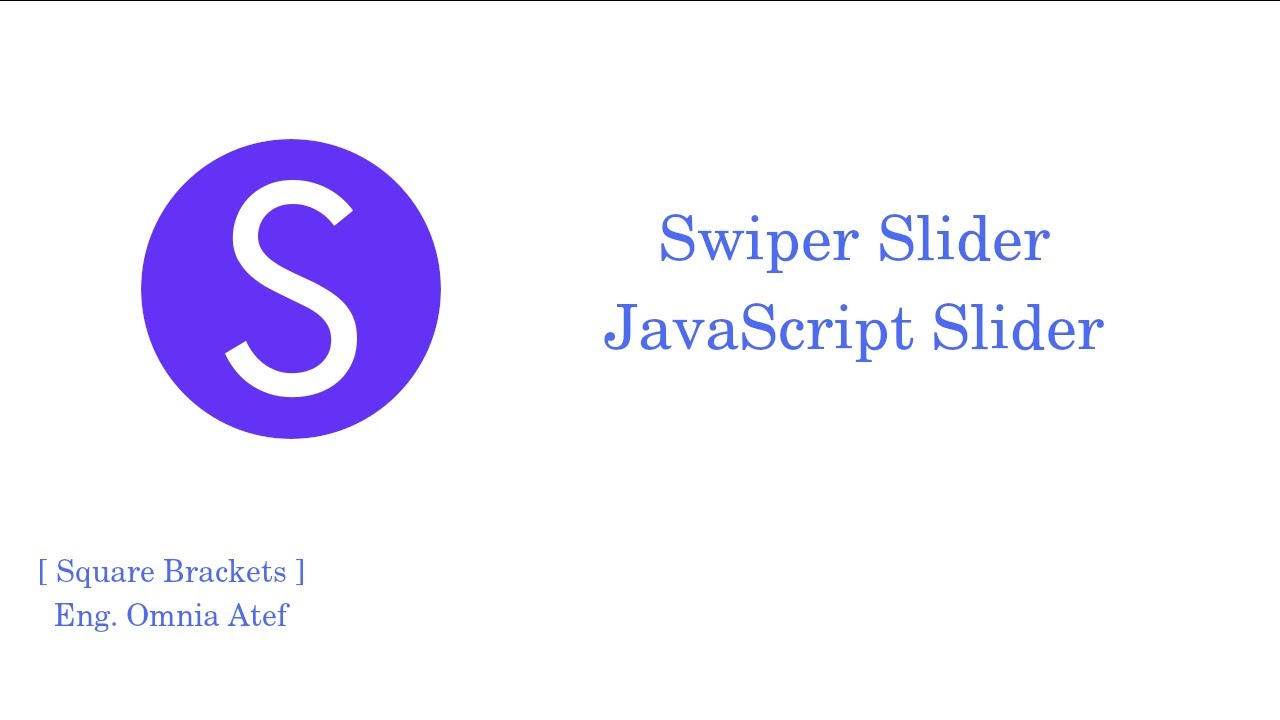The screenshot captures a focused element from a website against a clean, white background. Toward the middle-right of the image, there is prominently displayed text in a light blue font that reads "Swiper Slider" with a subheading "JavaScript Slider" just beneath it. To the left of this text, there is a conspicuous, large purple circle featuring a bold, white letter "S" at its center. 

In the lower left-hand corner of the screen, there is additional text in the same blue font but in a smaller size. This text reads "[square brackets]", with noticeable spaces between the "S" and the opening bracket, as well as the last "s" and the closing bracket. Directly beneath this text is a sequence of words that seem to be acronyms or shorthand: "ENG."—likely indicating 'English'—followed by "OMNIA" and "ATEF" as separate terms.

Additionally, the very top edge of the image is subtly marked by an ultra-thin black line, providing a slight boundary at the extreme upper limit of the screenshot.